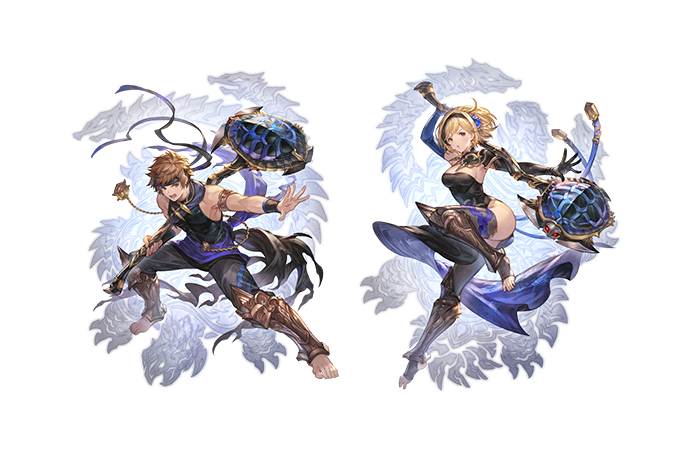This vivid and dynamic digital artwork, reminiscent of a DeviantArt piece, features two anime-style characters, a male on the left and a female on the right, engaged in a dramatic battle scene. The characters are poised in active fighting stances, each wielding a distinctive blue-and-black axe-like weapon. The heads of these axes resemble turtle shells, which are blue with black outlines. Both characters have fantasy-inspired costumes—sleeveless shirts, long pants (the male character also sports nightgreaves), and no shoes, embodying the vibrant colors of yellow, blue, gold, silver, and bronze. The male character's brown hair and the female character's yellow hair add a striking contrast to their attire. Behind them loom shadowy, multi-headed dragon figures, intensifying the epic fantasy atmosphere of the scene. Additionally, floating turtle shapes accompany both characters, reinforcing the fantastical elements of the artwork.